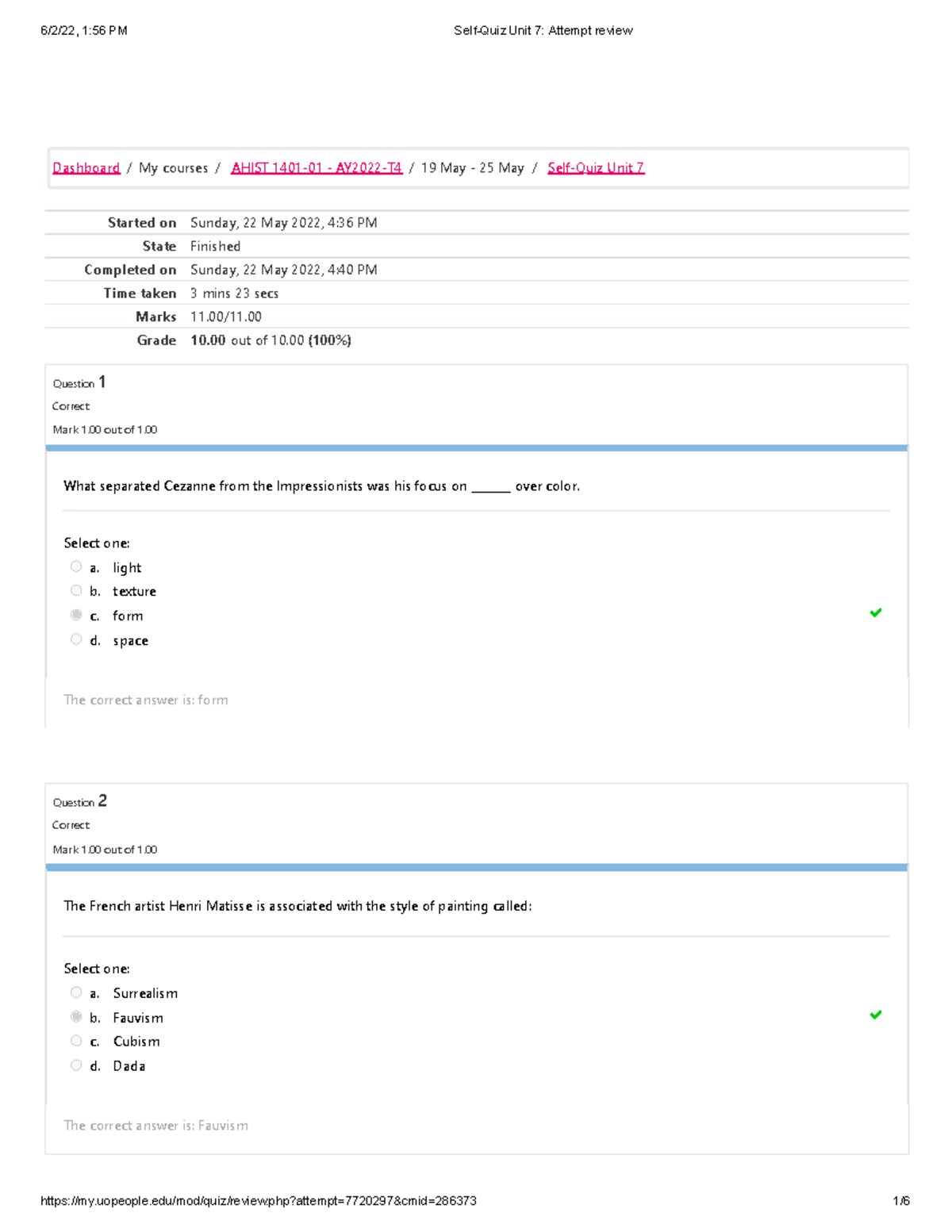This is an image of an online quiz attempt review from an educational platform. At the top center, the title "Self Quiz Unit 7 Attempt Review" is prominently displayed. On the left, the date and time "5/22, 1:56 PM," though slightly blurred, are visible. Adjacent to this, breadcrumb navigation lists "Dashboard / My Course / [additional information]," leading to the quiz timeframe "19 May - 25 May / Self Quiz Unit."

The document details the quiz's metadata including "Started On," "Completed On," "Time Taken," "Marks," and "Grade." Below these details, Question 1 is presented with a blue separator line. The question reads: "What separates Kazin from the Impressionists was his focus on space over color." The possible answers, labeled A through D, follow beneath the question. The correct answer, C, is highlighted in a gray shade.

Following a similar format, Question 2 is displayed, stating: "The French artist Henri Matisse is associated with the style of painting called:" with multiple-choice options listed below. Each question is structured consistently, facilitating clear and organized review of the quiz attempt.